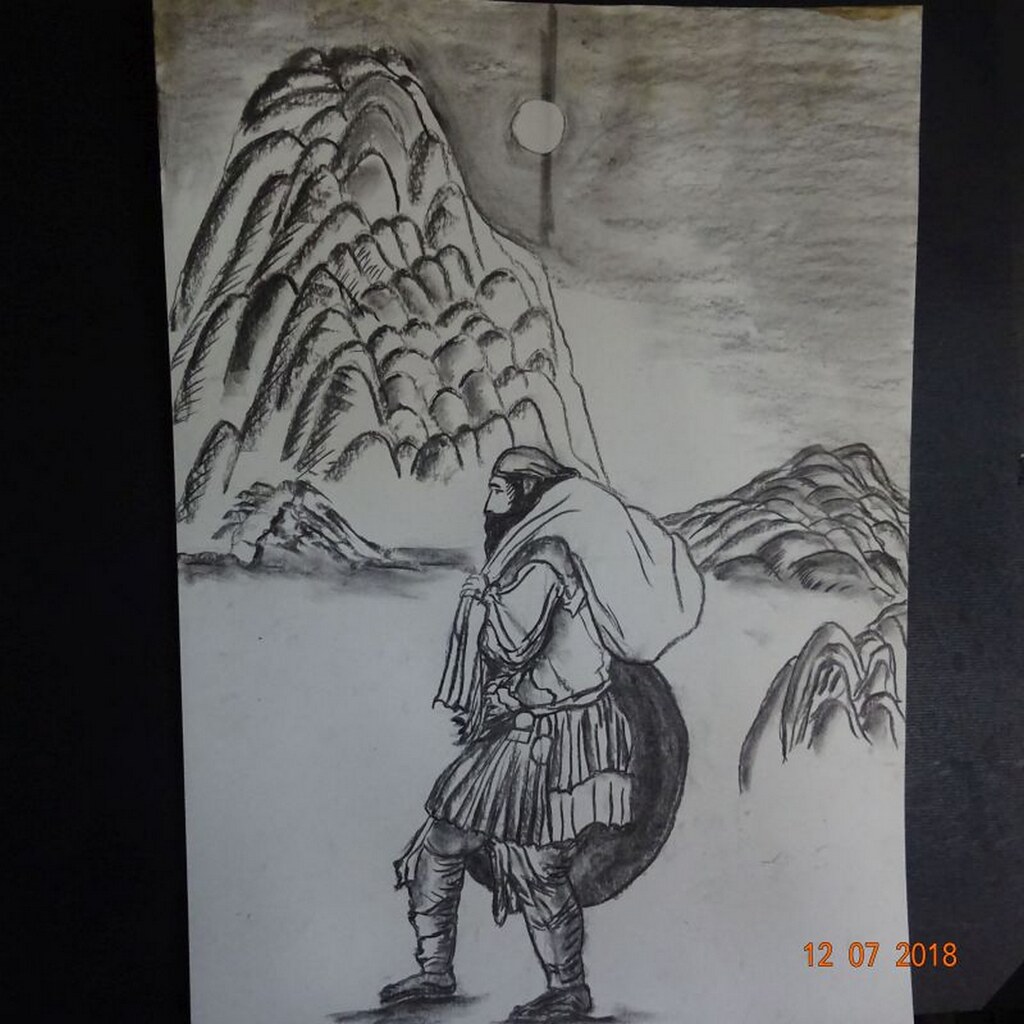In the image, there is a photograph capturing a detailed black-and-white sketch on white paper, which likely originated from a sketch pad. This sketch, executed with either a dark pencil or charcoal, depicts a bearded samurai with a long black beard and mustache. The samurai is dressed in attire reminiscent of medieval times, holding a shield in his right hand and a knapsack slung over his left shoulder. He appears to be walking in front of a mountainous backdrop. Specifically, there are three mountain-like structures; the tallest one is to the left, while the other two are smaller. A small, round white circle, likely the sun, is visible in the sky. The sketch is flanked by black vertical strips on both the left and right sides of the image. At the lower right corner, a red timestamp indicates the date 12-07-2018.